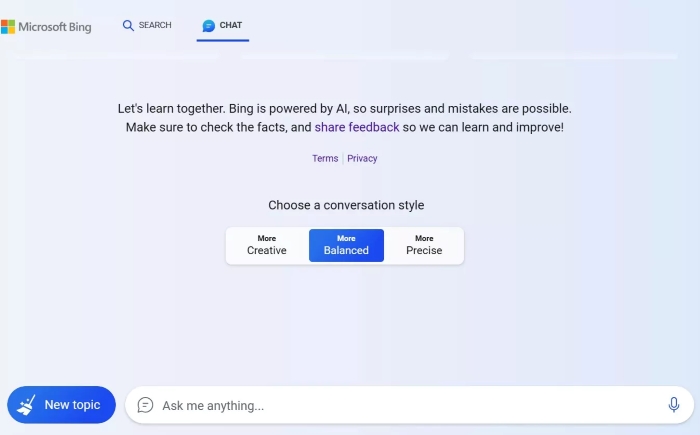The image presents the Microsoft Bing chatbot interface, featuring a clean, gradient background that transitions from very light gray in the lower right to light purple and then light blue towards the top left. In the top left corner, the iconic Microsoft logo is displayed, consisting of four small squares: red, green, blue, and yellow. To the right of the logo, the text "Microsoft Bing" appears in gray.

Next to this, a dark blue magnifying glass icon is followed by the word "SEARCH" in uppercase, black lettering. Adjacent to this, there is a blue chat bubble icon with white lines representing text, and to its right, the word "CHAT" is prominently displayed in bold, uppercase black letters, underlined in blue to indicate it is selected.

In the upper center of the page, a welcoming message reads: "Let's learn together. Bing is powered by AI, so surprises and mistakes are possible. Make sure to check the facts, and share feedback." The phrase "share feedback" is highlighted in dark purple, indicating it is a clickable link that has been accessed before. The message concludes with: "so we can learn and improve!"

Immediately below, in the same dark purple, the link text "Terms" is followed by a light gray line, then "Privacy." Further down, the text "Choose a conversation style" appears in black font. Three conversation style options are available: "Creative" on the left, "Balanced" in the center, and "Precise" on the right. The currently selected option, "Balanced," is highlighted in blue, while the other two options remain in white. Each option includes the word "More" in smaller, bold lettering at the top, followed by their respective descriptions ("Creative," "Balanced," and "Precise") in larger, non-bold text beneath.

The interface blends clean design with user guidance and interactive elements, underscoring Microsoft's commitment to a user-friendly AI experience.